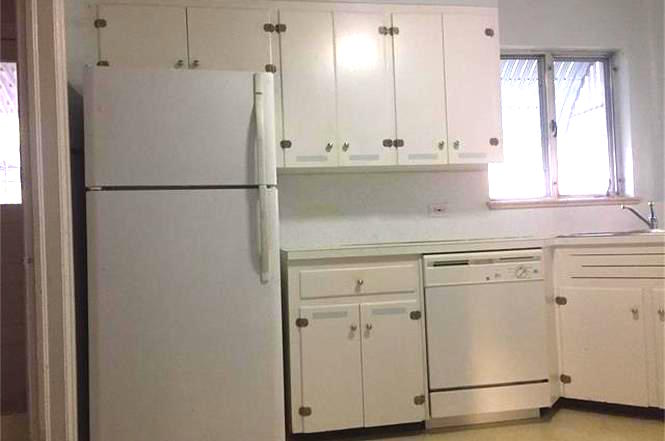The image depicts a pristine, all-white kitchen featuring various appliances and cabinetry. On the far left stands a tall, plain white refrigerator with a bottom fridge compartment and a top freezer section. Above the refrigerator are short white cabinets with metal hinges. Next to the fridge, moving right, are additional white, wall-mounted cabinets and a segment of countertop with more cabinets beneath, including a drawer. Adjacent to this area is a white dishwasher. The kitchen sink, equipped with a silver faucet, is located further to the right, set at a 45-degree angle from the other appliances. Above the sink is a two-panel window, brightly illuminated by sunlight, revealing a canopy or shading device outside. The floor appears slightly off-white, possibly covered with a rug. The entire aesthetic of the kitchen is emphasized by its uniform white color scheme, accented only by silver hardware and fixtures.